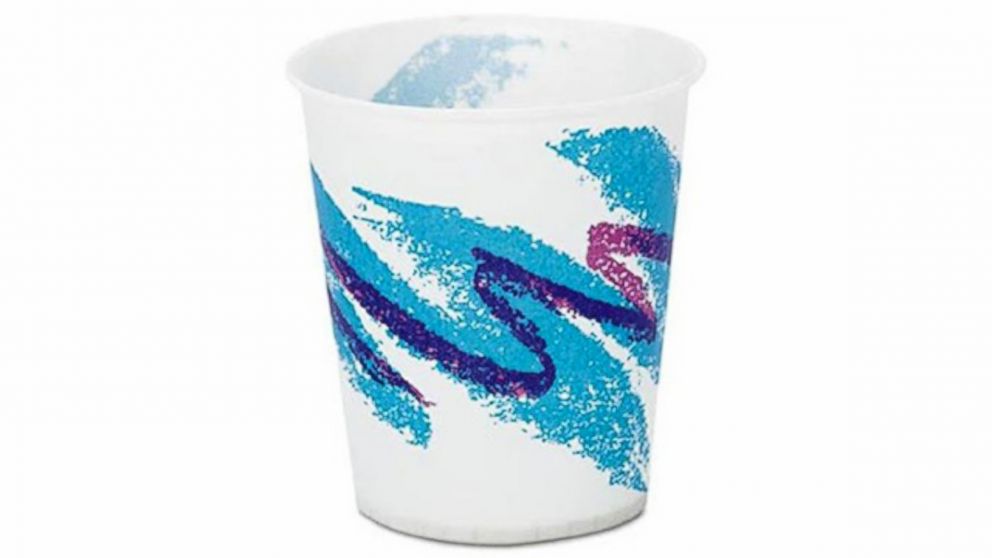This image showcases a classic, disposable paper cup commonly associated with ice cream parlors and reminiscent of designs from the 1990s. It is a white Dixie cup adorned with a distinctive, colorful pattern. The design features light blue swirls that resemble a paint-roller effect, with white speckles breaking through the blue, extending across the middle and veering out towards the sides. Intermingling with the blue swirls is a purple ribbon-like swirl, adding a layer of visual interest with its curved path. The cup stands upright in the photograph, perfectly centered, with its empty mouth clearly visible. The overall aesthetic gives off a nostalgic and vibrant feel, predominantly showcasing the light blue and purple colors against the white background. This disposable cup is typical of those used for serving ice cream in shops or for casual use at events, easily recognizable by its popular and enduring design.